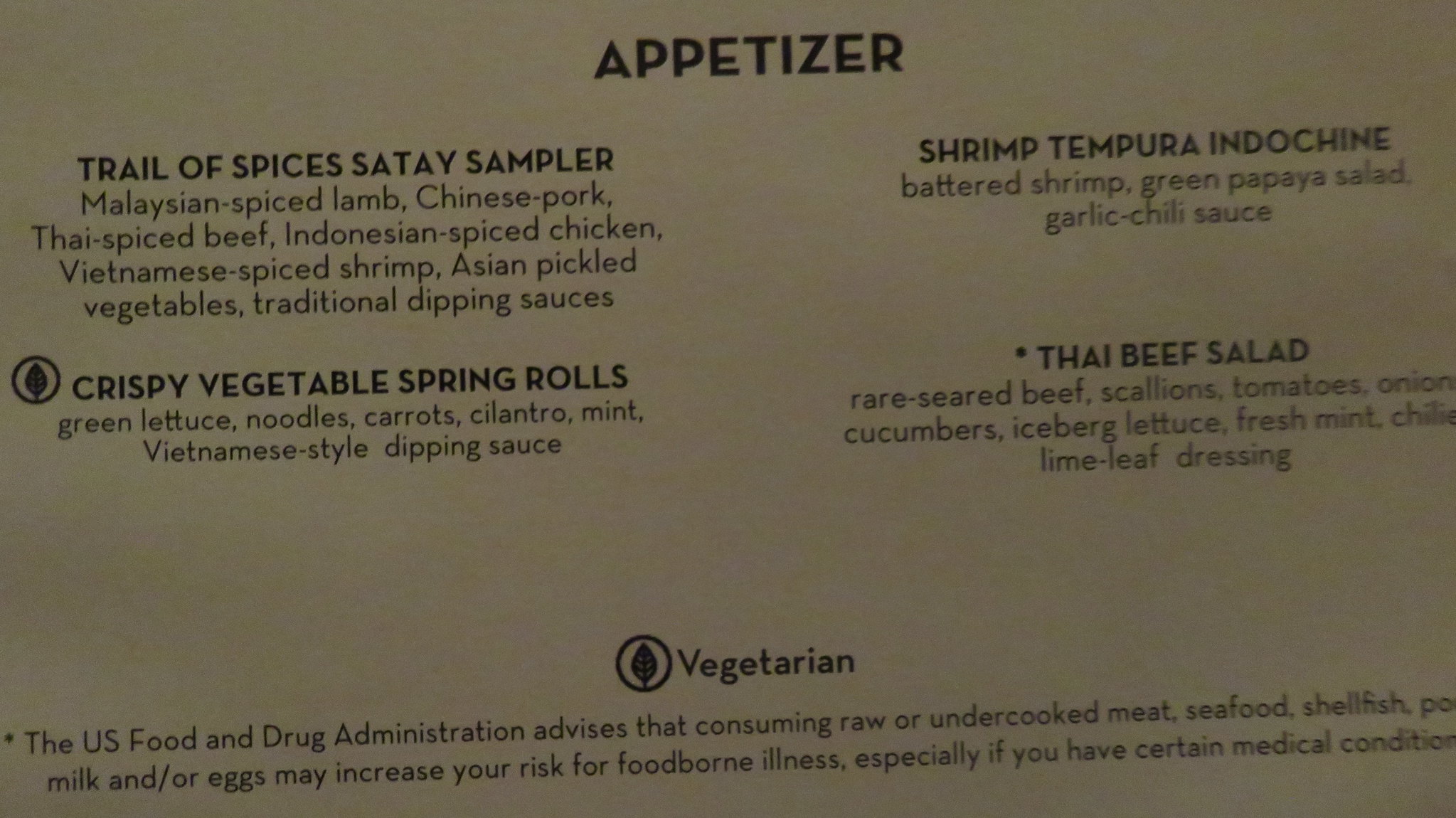The image depicts a black and white appetizer menu with a gray background and black text. At the top center, the title "APPETIZER" is prominently displayed in all capital letters. The menu is divided into four distinct appetizer options. On the top left, "Trail of Spices Satay Sampler" is listed, with an extensive description omitted for brevity. Below this on the left side, "Crispy Vegetable Spring Rolls" are described, featuring ingredients such as green lettuce, noodles, carrots, cilantro, mint, and Vietnamese-style dipping sauce, alongside a vegetarian symbol represented by a circle with a leaf. On the top right, "Shrimp Tempura Indochine" is featured, detailing battered shrimp, green papaya salad, and garlic chili sauce. Just below this on the right side, "Thai Beef Salad" is described with rare seared beef, scallions, tomatoes, onions, cucumbers, iceberg lettuce, fresh mint, and lime leaf dressing, accompanied by an asterisk. At the bottom of the menu, an asterisk explains that the U.S. Food and Drug Administration advises that consuming raw or undercooked meats, seafood, shellfish, poultry, milk, or eggs may increase the risk of foodborne illness, especially for individuals with certain medical conditions. Detailed descriptions for each dish are provided under their respective titles.